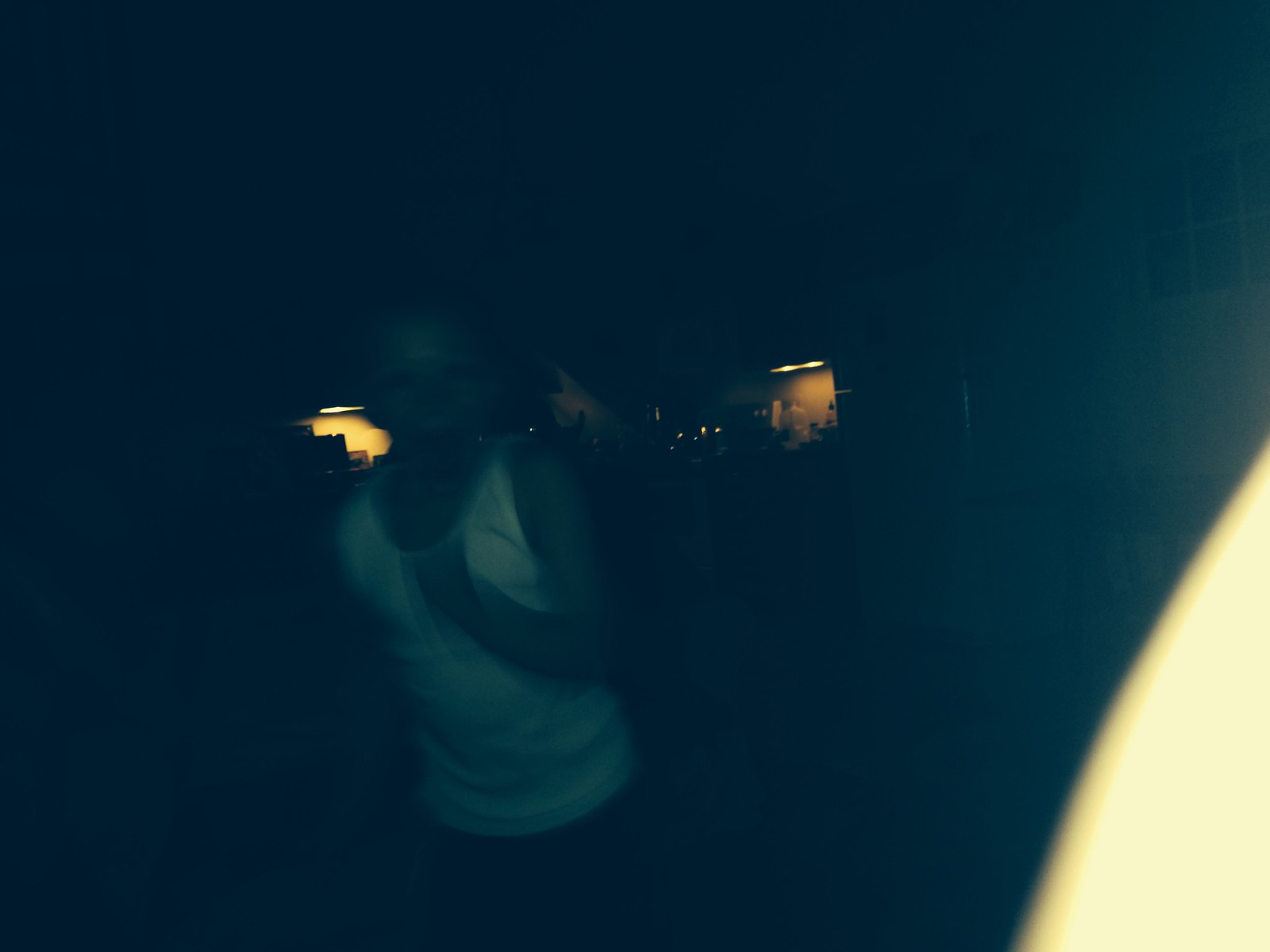In the image, we see a very dark, nighttime scene. The central focus is a light-skinned, hairless, male figure wearing a white tank top and black pants, moving towards the camera. His left arm is raised to his chest in a running or fast-walking pose. The face is difficult to make out, but there's a suggestion of a surprised or unsettling expression. To the right side and top of the image, there's a distinct whitish-colored building with a multi-pane window divided by white pillars, and an orange light emanating from it. In the bottom right corner, a yellowish flash is visible, likely an obscuring finger of the person taking the photo. The overall atmosphere is eerie, comparable to a ghostly apparition, adding to the unsettling feeling of the image.